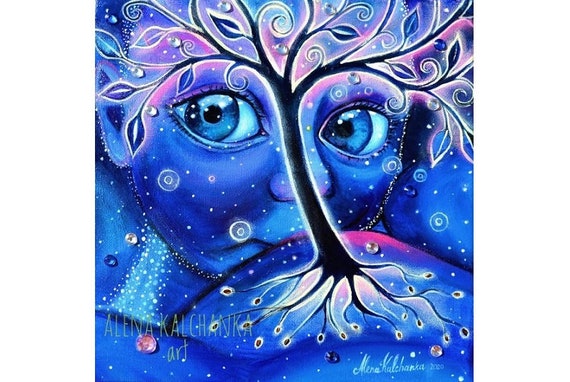This artwork by Alina Kalchanka, created in 2020, intricately combines surrealism with a dreamlike aesthetic. Dominated by shades of blue with subtle hints of white and pink, the painting features a large, serene face with strikingly big blue eyes that exude a sense of ethereal happiness. In the foreground, a tree with illuminated roots emerges from a mound of earth, its trunk and branches extending upwards and aligning with the features of the face behind it—intersecting with the nose, forehead, and eyes. The surreal landscape is accentuated by stars that twinkle within the face, blending celestial elements with the earthly scene. The piece is signed "Alina Kalchanka Art" on the bottom left and "Mina Kalchanka 2000" on the bottom right, adding a personal touch to this mesmerizing and harmonious composition.